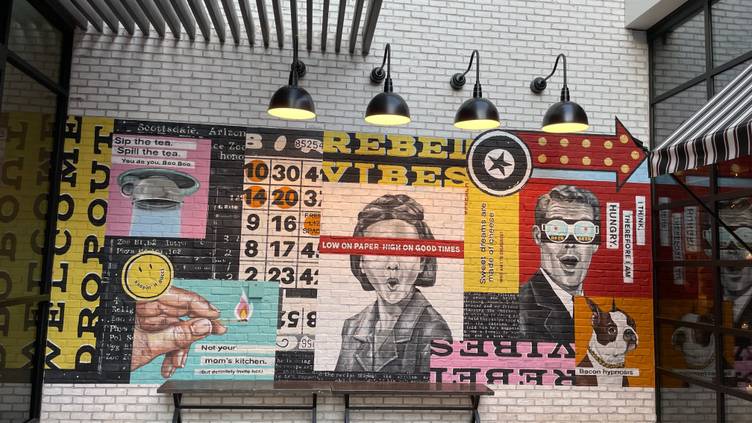The image depicts a brick wall painted white, adorned with several murals and illuminated by four black lamps hanging from the top. Dominated by eclectic artwork, the wall features multiple illustrations and text: in the upper left, a pink section with a picture of a tea kettle and the phrases "sip the tea," "spill the tea," and "you do you, boo boo." At the top, a yellow mural proclaiming "Rebel Vibes" includes a depiction of a person with a red banner over their eyes and the text "low on paper, high on good times." There’s also a painting of a man wearing blue glasses with the humorous caption, "I think therefore I am hungry," along with a red arrow pointing to the right. In the bottom right corner, there’s an orange section portraying a dog with the phrase "bacon hypnosis." Additional elements include windows and a canopy to the right of the wall, likely covering an entryway, and two small benches positioned below the murals. This detailed and vibrant depiction suggests a unique and artistic space, likely a coffee shop named Rebel Vibes.